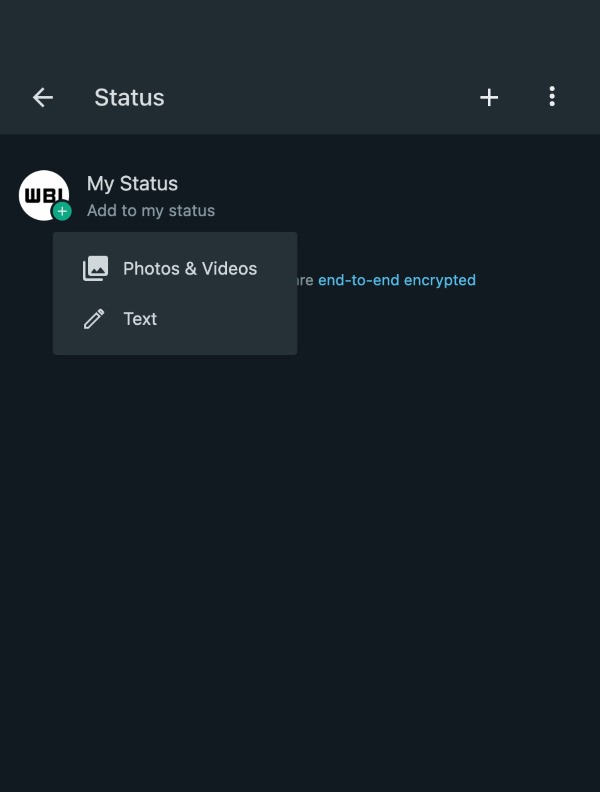This image appears to be a screenshot of a phone interface, possibly from a messaging app. The screen transitions from a dark gray at the top to a pitch-black color towards the bottom. 

At the top in the dark gray section, there's an arrow pointing left labeled "Status". To the right of this, there is a plus sign followed by three vertical dots, likely representing a menu or options.

In the black section below, a white circle containing the letters "WBI" is prominently displayed next to the words "My Status." Beneath that, in muted gray text, it reads "Add to my status."

A pop-up box overlays this area, containing icons and text. The first icon shows two overlapping rectangles, symbolizing "Photos and Videos," and the second icon, a pencil, represents "Text." Below these icons, partially obscured, is gray text displaying the letters "URE." In teal blue text, the image notes, "End-to-end encrypted."